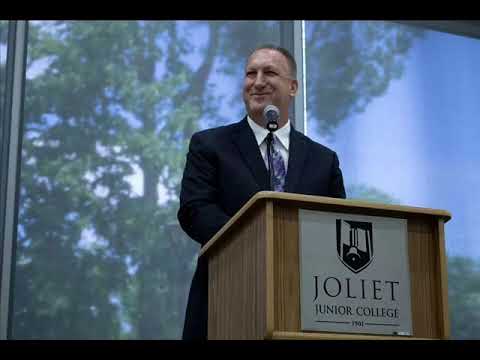In this image, a well-dressed man is standing at a wooden podium with a microphone, delivering a speech at Joliet Junior College. He is wearing a dark suit, a white shirt, and a distinctive purple tie, with short hair and a beaming smile. The podium bears an emblem that reads "Joliet Junior College 1901," indicating the college setting. The background features two large windows framed with beams, revealing a scenic view of lush green trees with leaves, a blue sky, and scattered white clouds. The overall setting suggests a bright day outside, although the event itself appears to be indoors. The colors in the image include the brown of the wooden podium, the silver and blue of the Joliet College signage, the black and gray of the microphone, the black suit, the white shirt, the purple tie, the man's skin tone, the blue sky, and the green trees. The man is centered in the image, making him the focal point, possibly indicating he is a notable speaker such as a university professor, president, or a guest lecturer.